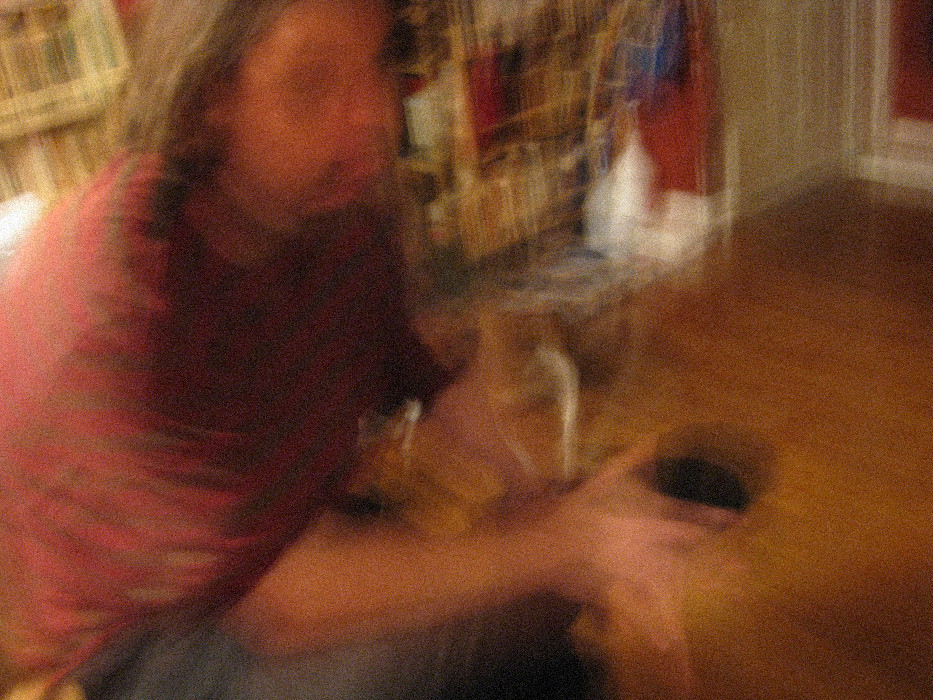The image depicts an extremely blurry photo of a white, middle-aged man with long brown hair, sitting down on furniture placed on a brown wood grain floor. The man, who appears to be holding a black drink in a cup with his right hand, is dressed in a red short-sleeved shirt and blue jeans. Behind him, there's a shelf that holds either books or DVDs, and a second shelf partially obscures his face. The background features various elements, including a little bit of a red wall with white trim, an out-of-focus white door, and possibly some red, blue, and white cloth hanging from one of the shelves. The overall scene is chaotic and detailed, yet highly obscured due to the extreme blurriness of the photo.